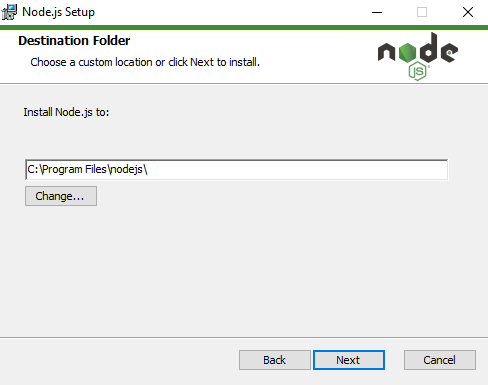A screenshot of the Node.js setup wizard is displayed, featuring a prominent white pop-up box with a computer icon and the title "Node.js Setup" at the top. The top right corner includes a minus sign, a gray box, and a gray 'X'. Below, a thin green progress line is visible.

The main body of the pop-up contains instructions for the installation process. In red and black text, it states: "Choose a custom location or click next to install." The Node.js logo, comprising a stylized "N" with a person icon, a green "O," black "D" and "E," and a small circle containing "JS," is prominently featured.

Further down, the destination folder path is displayed: "C:\\Program Files\\nodejs\\" in a white box. Options to change this path, go back, proceed to the next step, or cancel the installation are presented in gray boxes, with the "Next" button highlighted in blue. The text is large and user-friendly, ensuring excellent visual clarity and ease of reading. No other objects or text are present in the image.